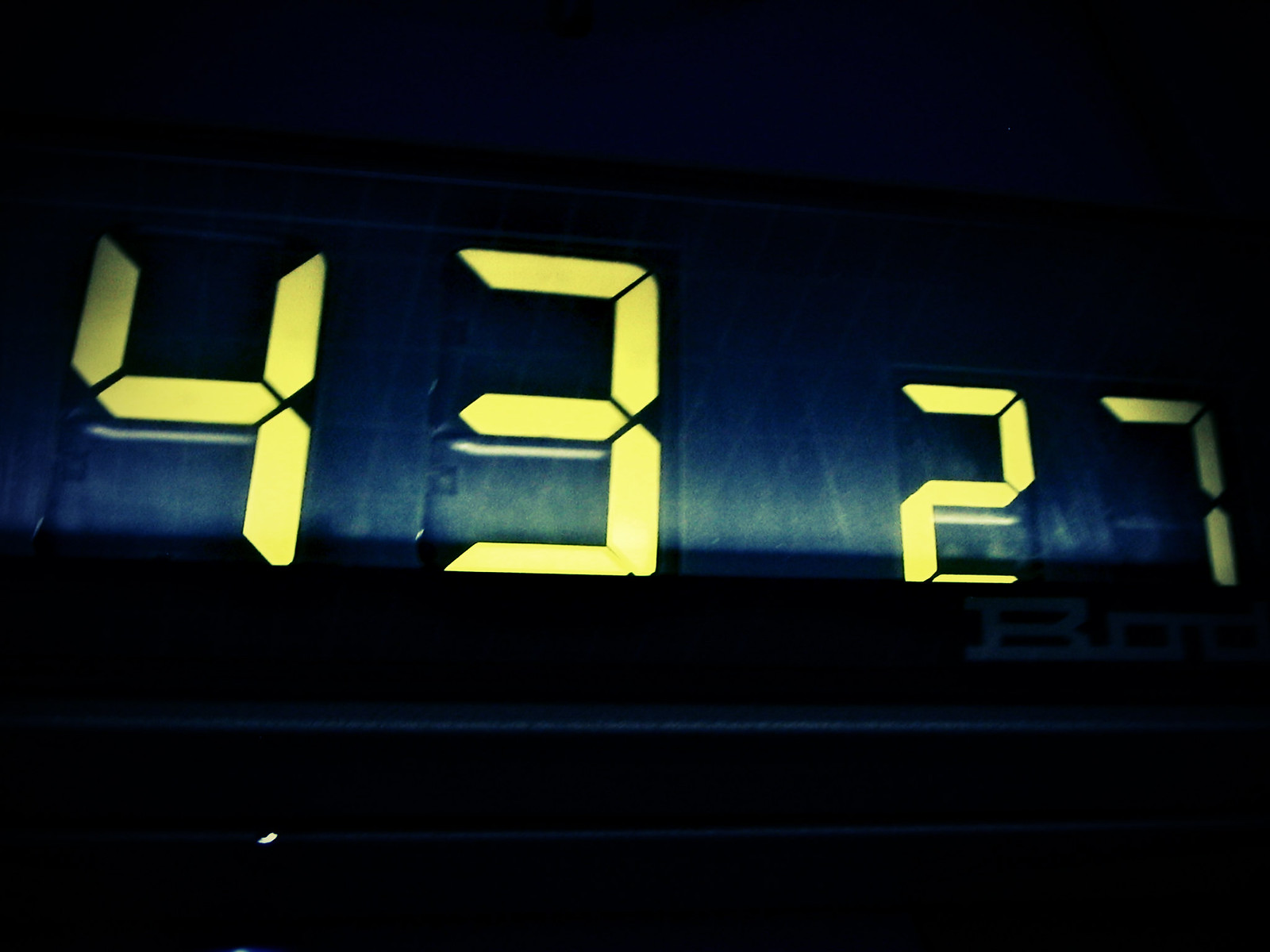This close-up color photograph captures the digital display of an alarm clock in low light. Dominating the image, a large yellow "43" stands prominently to the left, while to its right, a smaller "27"—about two-thirds the size of the "43"—is displayed. Both sets of numbers are in a digital font characteristic of alarm clocks. The background is predominantly a dark blue-gray, with a faint lighter area in the middle, slightly illuminated to enhance the visibility of the numbers. Below the "27," the beginning of a brand name or word is visible, starting with a capital "B" followed by two lowercase "o's" in gray lettering. The overall lighting is dim, giving the scene a somewhat sketchy and mysterious vibe, with detailed lines clearly visible despite the low light.